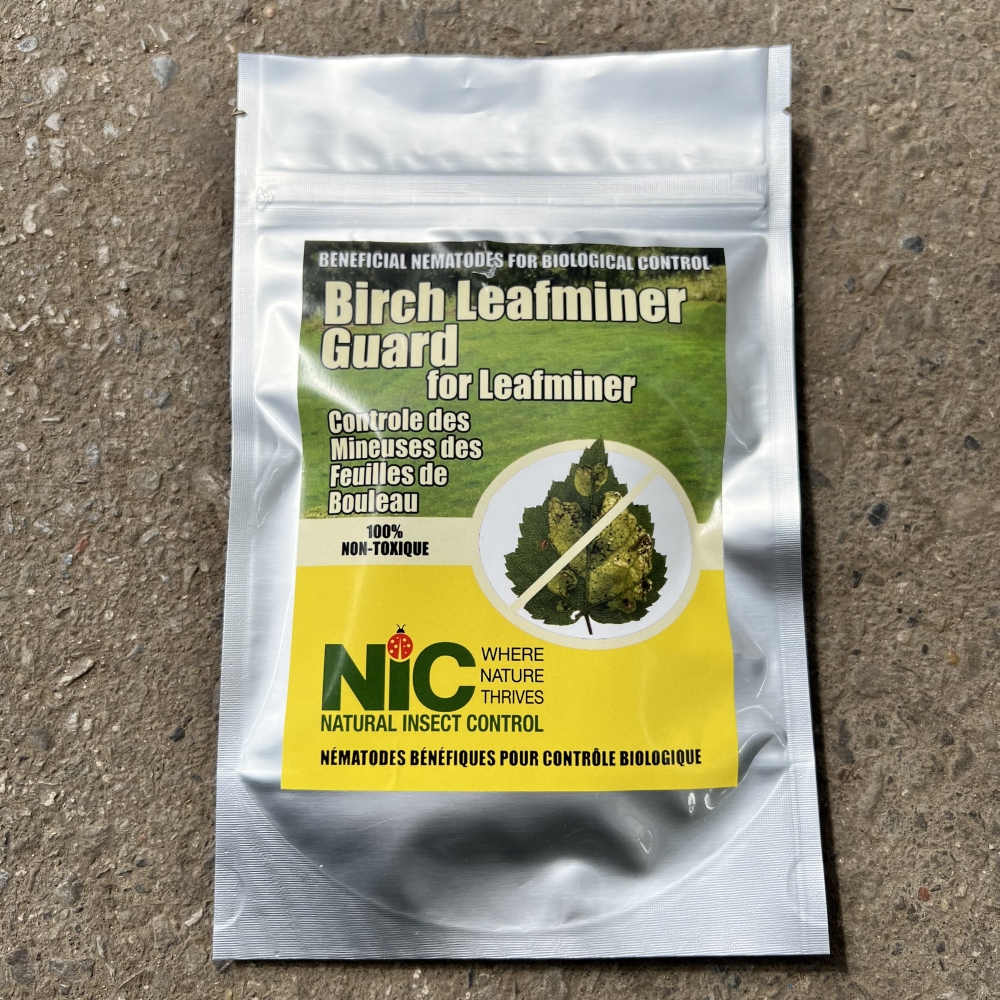This image depicts a silver, shiny, Ziploc-style bag against a gravel or stone-like surface. The bag features a large rectangular label. At the top, the label reads "Beneficial Nematodes for Biological Control." Below this, it states "Birch Leafminer Guard for Leafminer" alongside the French translation "Contrôle des Menus de Faisu de Belleu." Further down, the text in French reads "100% Non-Toxique." An image of a discolored leaf with a cross through it signifies its pest control purpose. Underneath, the text "N.I.C." appears in green with a red ladybug on the "I," followed by the slogan "Where Nature Thrives" and "Natural Insect Control." The overall aesthetic points to a product designed to protect plants from harmful insects in a non-toxic, eco-friendly manner.